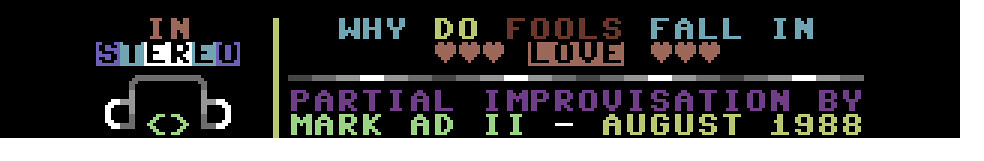The image is a narrow, horizontal rectangle that appears to be a section of a digital screen, possibly from a jukebox or a cell phone display. The background is completely black. Starting from the left, there are the capital letters "IN" in brown, followed by the word "STEREO" in a gradient of purple, blue, white, then blue, and purple letters. Below this, a small graphic resembling a robot or a face with a green image in the center is present within a curved rectangle. There’s a yellow vertical line or bar adjacent to this graphic that doesn’t extend to the top of the black background.

On the right side, the words "Why do fools fall in love?" are written across the top of the image with each word in different colors: Y in light blue, DO in yellow, FOO in light purple, LIGHT blue for FOOLS, light blue for FALL, and light blue again for IN. There are three red hearts on either side of the word "LOVE," which is written within a red rectangle. Below this text, a white horizontal line bordered by alternating shades of gray stretches across the width of the image.

Further down, the phrase "Partial Improvisation" is written in purple letters, followed by "by MARK82 - AUGUST 1988" in green letters. The entire setup is on a continuous black background, making the colorful fonts and graphics stand out.